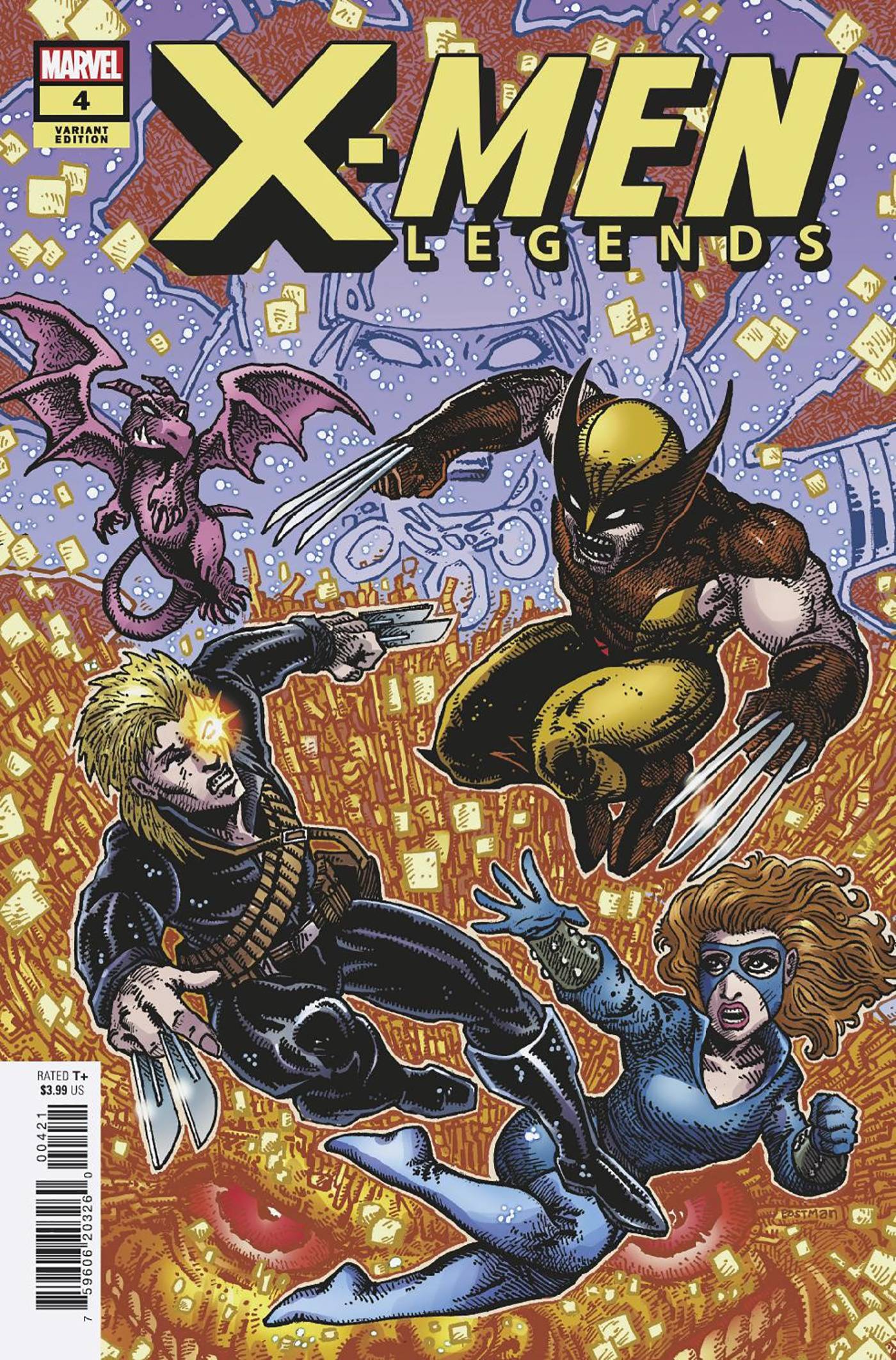The vertical rectangular comic book cover features bold, large yellow letters at the top spelling "X-Men," with "Legends" in smaller yellow text beneath it. A blue background with various objects flying around transitions into vibrant hues of orange, red, and yellow in the lower part of the image. Dominating the scene are three distinct superheroes.

At the center, Wolverine is airborne, knees bent, clad in yellow tights and helmet, a brown chest piece, and brown gloves. His three long, silver claws extend from each hand, and he has distinctive brown "wings" on either side of his face. His mouth is open in a fierce expression.

Below Wolverine is a woman in a light blue spandex suit with a matching mask. She has long, flowing blonde hair and is reaching up towards Wolverine. 

Beside her is a man dressed in black spandex, sporting shaggy blonde hair with a glowing eye emitting a muzzle flash. He has two blades extending from each finger.

An enormous, menacing creature with a large orange face, evil red eyes, and yellowish teeth dominates the lower half of the cover. Its orange skin has strands and yellow squares throughout, adding to its chaotic appearance. A purple dragon can be seen behind the characters, adding more layers to the intense scene.